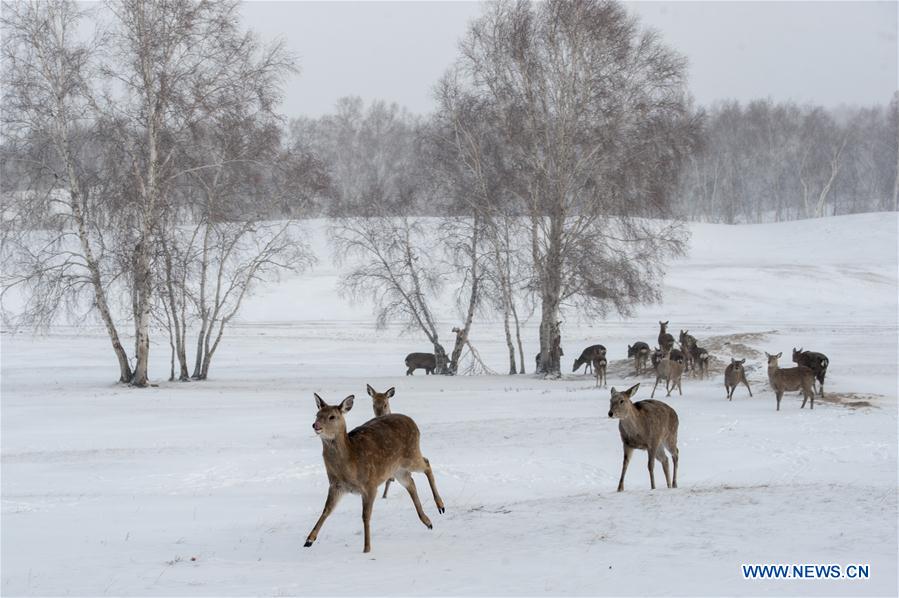This is a detailed nature and wildlife photograph of a snowy field taken from www.news.cn, as indicated by the blue text in the bottom right corner. The image captures a serene, winter scene featuring a herd of deer, probably white-tailed or mule deer, grazing near scattered hay. The field is expansive and slightly rolling, providing a crisp white backdrop that enhances the vivid brown tones of the deer. None of the deer, which are mature and lack spots, have visible antlers. Most of them are facing the camera, with three prominently moving towards the photographer. In the foreground, there are a few bare-leaf deciduous trees with white bark, likely from the Aspen family. The background is lined with more deciduous trees, equally barren of leaves, under a gray and overcast sky, adding to the wintery ambiance. There are no buildings in sight, emphasizing the untouched and tranquil nature of the landscape.